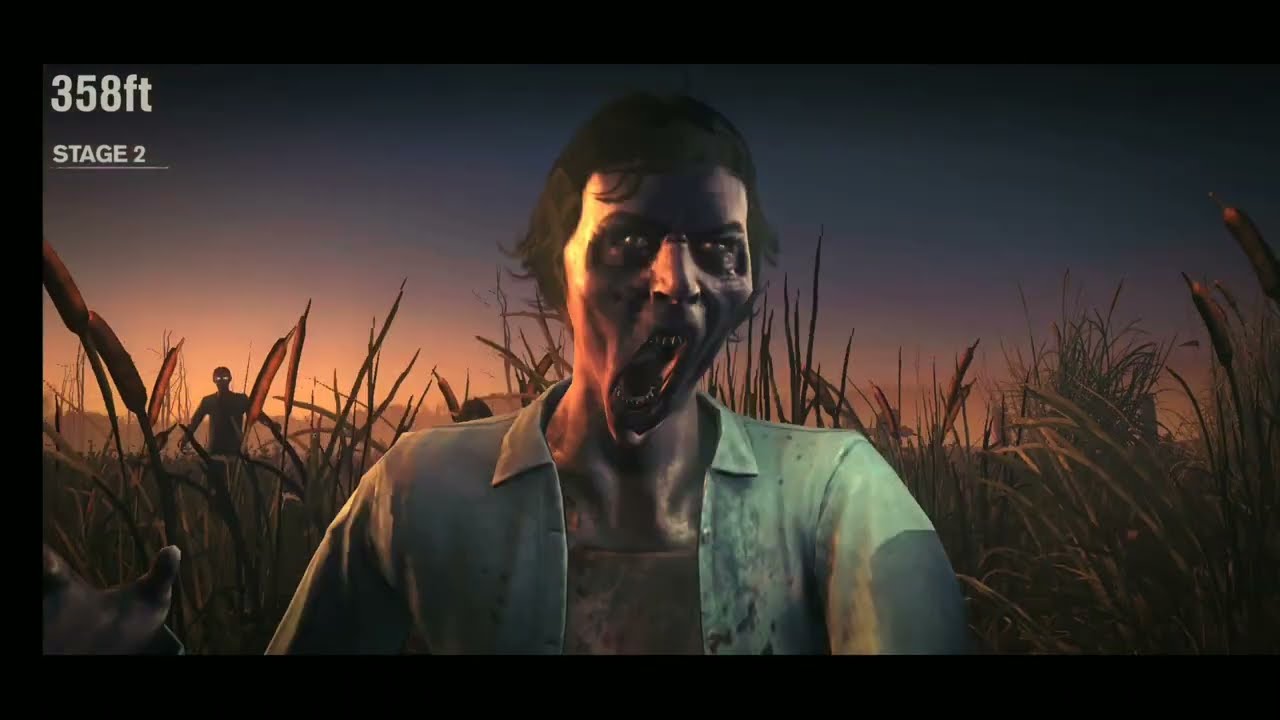The image appears to be a digitally created scene from a video game, showcasing a night setting in a field or cornfield with tall plants. The central figure in the image is a zombie-like creature, wearing a green shirt. Its face is grotesquely distorted with unnaturally elongated and sharp teeth, wide hollow eyes that look possessed, and a mouth opened as if screaming. Its skin appears to be burned or decayed, giving it a shiny brown texture. Behind the central figure stands another zombie, recognizable by its glowing white eyes and a blood-stained, open shirt. The background is dusky with a dark navy blue sky, indicating that nighttime approaches. The upper left corner of the image features text reading "358 feet" and "Stage 2," hinting at the game's progress. This scene sets a tense atmosphere as the zombies appear to be poised to attack, capturing a quintessentially terrifying moment in the game.